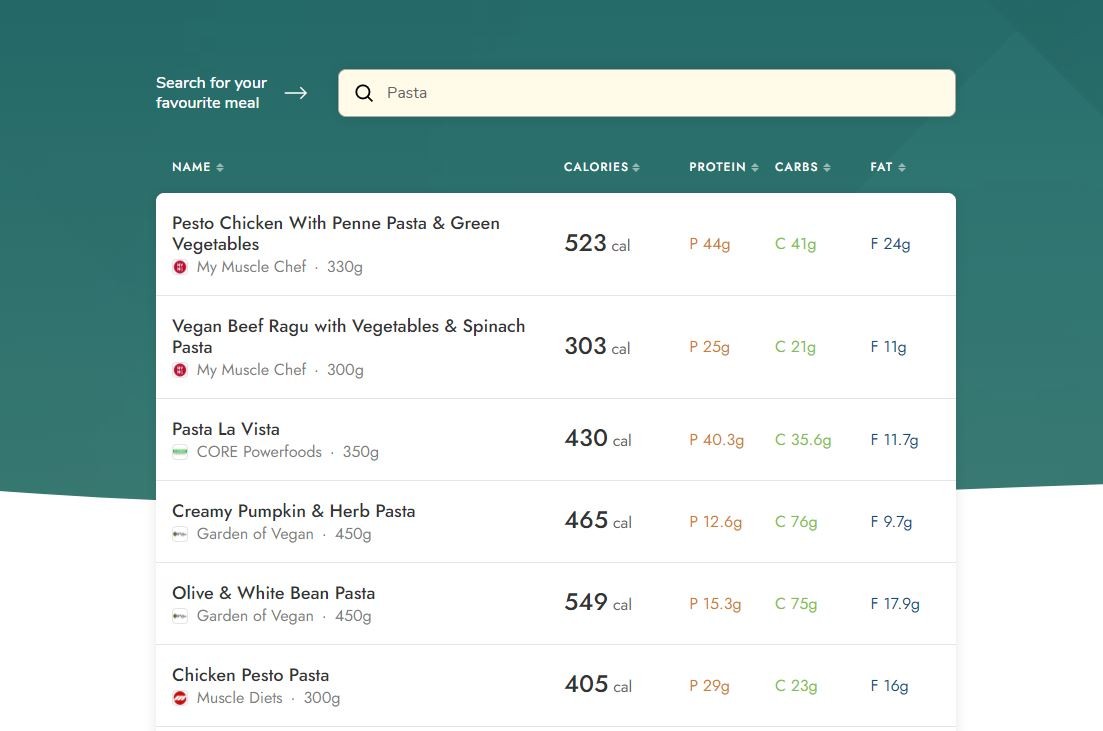The image displays a web interface dedicated to meal search and nutritional information. At the top, a prompt encourages users to "Search for your favorite meal," accompanied by an arrow pointing to a search bar where the term "pasta" is entered. Below the search bar, the interface is organized into columns with headings in uppercase white text: "NAME," "CALORIES," "PROTEIN," "CARBS," and "FAT."

For instance, under the "NAME" column, there are detailed examples such as:
1. **Pesto Chicken with Penne Pasta and Green Vegetables (My Muscle Chef, 330 grams)**  
   - **CALORIES:** 523
   - **PROTEIN:** 44 grams
   - **CARBS:** 41 grams
   - **FAT:** 24 grams

2. **Vegan Beef Ragù with Vegetables, Spinach, and Pasta (My Muscle Chef, 300 grams)**  
   - **CALORIES:** 303
   - **PROTEIN:** 25 grams
   - **CARBS:** 21 grams
   - **FAT:** 11 grams  
   (this entry is marked with a red dot)

3. **Pasta La Vista (Core Power Foods, 350 grams)**  
   - **CALORIES:** 430
   - **PROTEIN:** 40.3 grams
   - **CARBS:** 35.6 grams
   - **FAT:** 11.7 grams

Each meal listed provides comprehensive nutritional data, helping users make informed dietary choices.